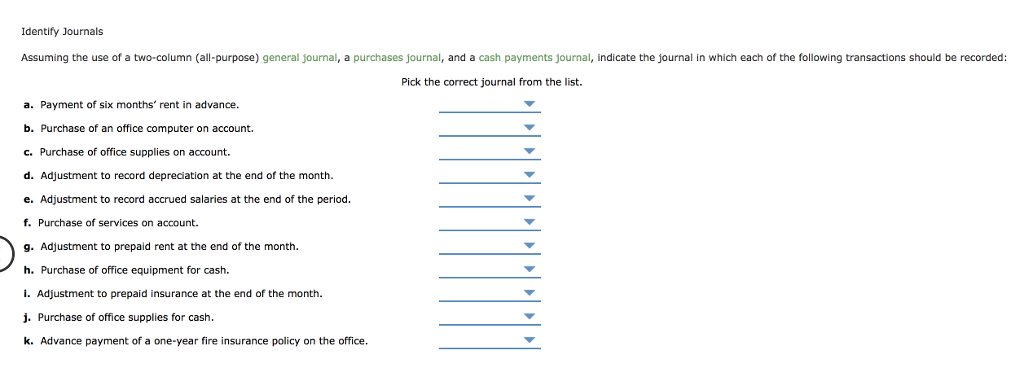The image is a detailed screenshot from a computer displaying a segment of a journaling and accounting software interface. At the top left corner, the header reads "Identified Journals." Beneath this, an instructional text is present, stating: "Assuming the use of two-column parentheses all-purpose general journal, purchase journal, and cash payments journal, indicate the journal in which each of the following transactions should be recorded."

The instructional text is color-coded to distinguish between the different types of journals: general journal, purchase journal, and cash payments journal. 

Below this instructional section, there are rows labeled A through K. Each row features a transaction description followed by a dropdown menu, allowing users to select the appropriate journal for recording. The transactions listed are as follows:
- A: Payment of six months rent in advance.
- B: Purchase of an office computer on account.
- C: Purchase of office supplies on account.
- D: Adjustment to record depreciation at the end of the month.
- E: Adjustment to record accrued salaries at the end of the period.
- F: Purchase of services on account.
- G: Adjustment to prepaid rent at the end of the month.
- H: Purchase of office equipment for cash.
- I: Adjustment to prepaid insurance at the end of the month.
- J: Purchase of office supplies for cash.
- K: Advance payment of a one-year fire insurance policy on the office.

At the very top of the dropdown section is the prompt: "Pick the correct journal from the list." This prompt reminds users to choose between the three available journals: general journal, purchase journal, and cash payments journal for each transaction type.

The interface is likely used for educational or professional purposes to teach or facilitate the correct categorization of financial transactions into their respective journals.